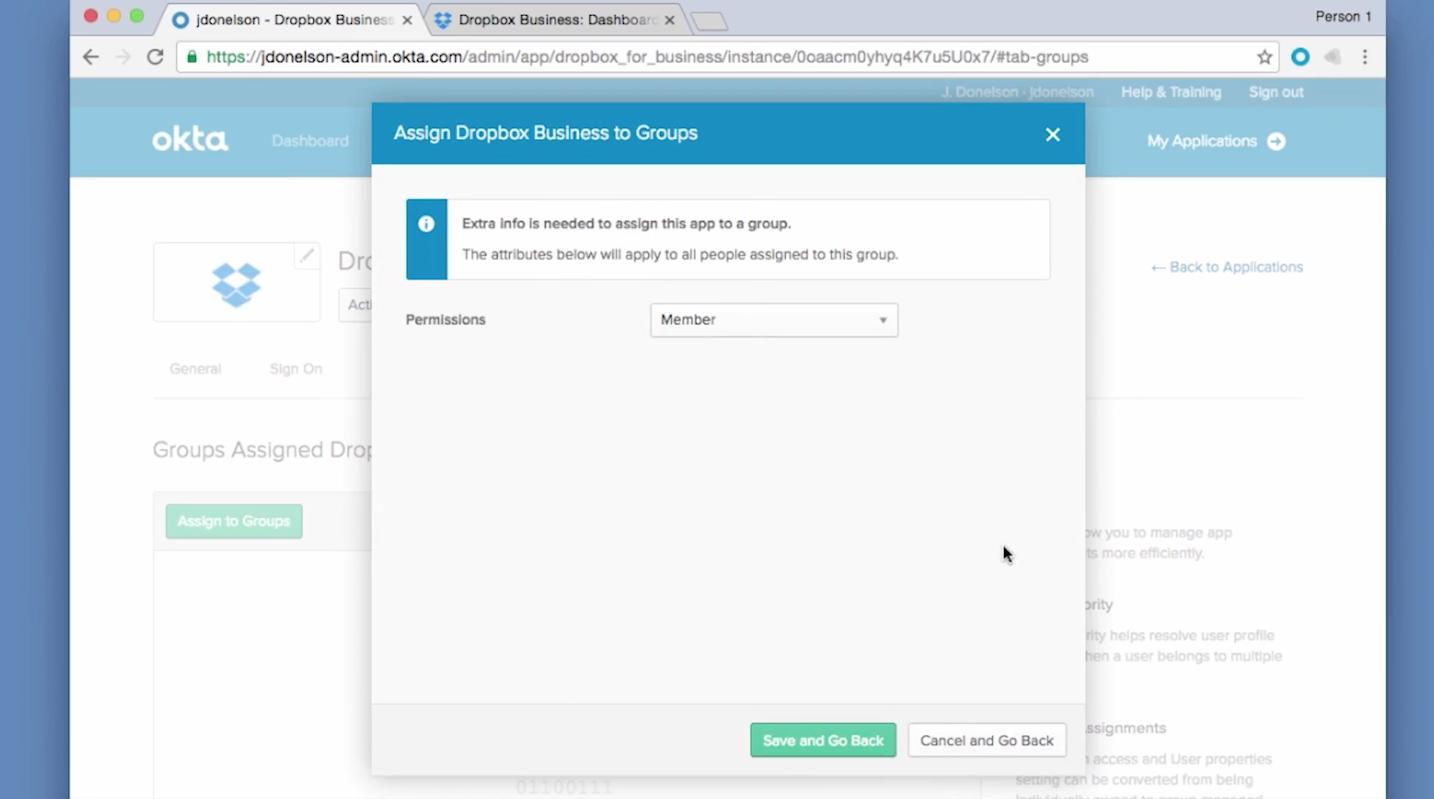A detailed screenshot of the J Donaldson admin website, accessible via jdonaldson-admin.okta.com, displayed within a web browser. The website showcases an interface dominated by blue hues. The entire header, as well as the side panels on both the left and right, are highlighted in blue. The main content area displays a dropdown menu titled "Assign Dropbox Business to Groups," indicating additional information is required to assign the application to a specific group. The permissions setting visible in the screenshot is configured to "member."